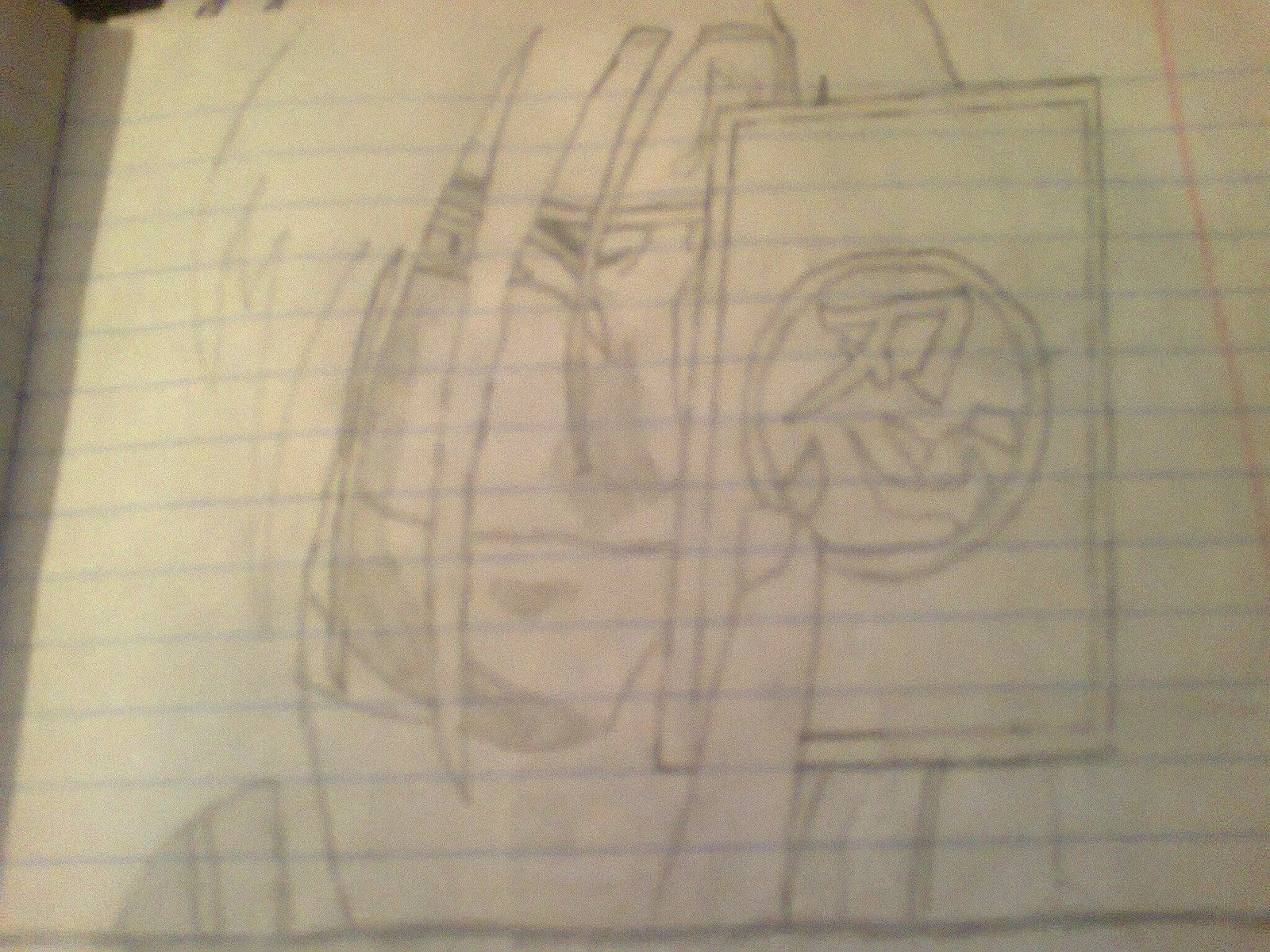The image is a photograph of a piece of lined notebook paper, featuring horizontal blue lines and a vertical red line on the right side. The paper bears a black pencil drawing, executed in a somewhat crude, anime-inspired style. The drawing depicts the close-up face of a person with long, spiky hair that obscures most of their visible eye, tapering sharply at the chin—characteristic of anime artwork. Prominently displayed in the foreground, a hand is seen holding a rectangular card with symmetrical borders. The card, detailed with an unrecognized symbol and possibly foreign characters, is positioned close to the face, drawing attention to the intricate designs within a central circle.